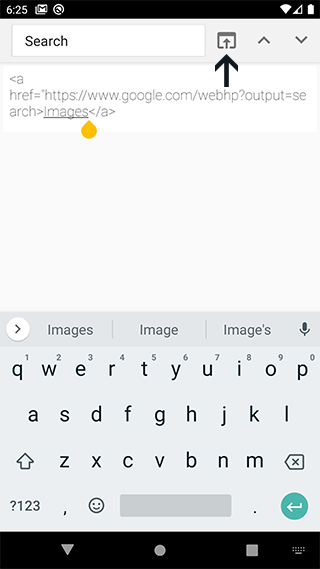This image displays a screenshot taken from someone’s cell phone, showcasing a list interface. At the top of the phone screen, there is a slim black rectangle that frames the display, indicating it is 6:25. Adjacent to the time, several icons are neatly aligned, including a picture icon, a circle icon, a Wi-Fi signal indicator, a triangle, and a fully charged battery symbol filled in with white.

Directly beneath these icons, a search bar is prominently positioned with an adjacent upload button, identified by an upward-pointing arrow likely added to highlight the button's function. Beside the upload button, there are up and down navigation buttons.

In the central section of the screen, some HTML code is visible, specifically: `<a href="https://www.google.com/webhp?output=search">images</a>`. A yellow pin, resembling a circular marker, points directly at the word "images" within this code.

The middle area of the screen remains blank, displaying a solid black background. The bottom of the image shows a visible keypad, suggesting that the user is in a text entry mode, ready to type.

The overall composition of the image captures a moment where someone is potentially illustrating the use of an upload button on a phone with annotations for instructional purposes.